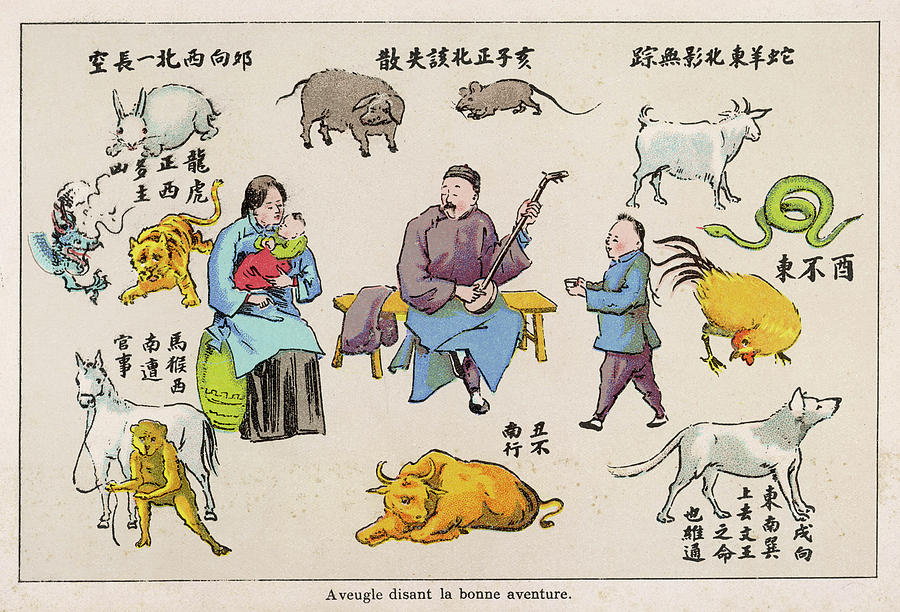The artwork is an old illustration on light tan paper, depicting an array of animals and a family scene. Animals such as a rabbit, rat, goat, cow, sheep, pig, cat, dragon, horse, bull, wolf, chicken, snake, tiger, and mouse are depicted, each associated with Chinese or Japanese characters. In the center of the image, a family scene unfolds: a man wearing a gray top, a blue bottom, and a black hat sits on a wooden bench playing an instrument resembling a mandolin or banjo. To his left is a woman in a blue top and gray bottom, sitting on a green pot and holding a baby dressed in a green top and red bottom. To the man's right is a shorter figure, possibly a child or young man, dressed similarly in a blue top and gray pants, walking towards the man with a cup or bowl. Surrounding this familial scene, the animals are illustrated in a hand-drawn, cartoony style with corresponding Chinese zodiac representations. The bottom of the illustration features a French caption, "A Vogue Descente La Bonne Adventure," suggesting a theme of good adventure.